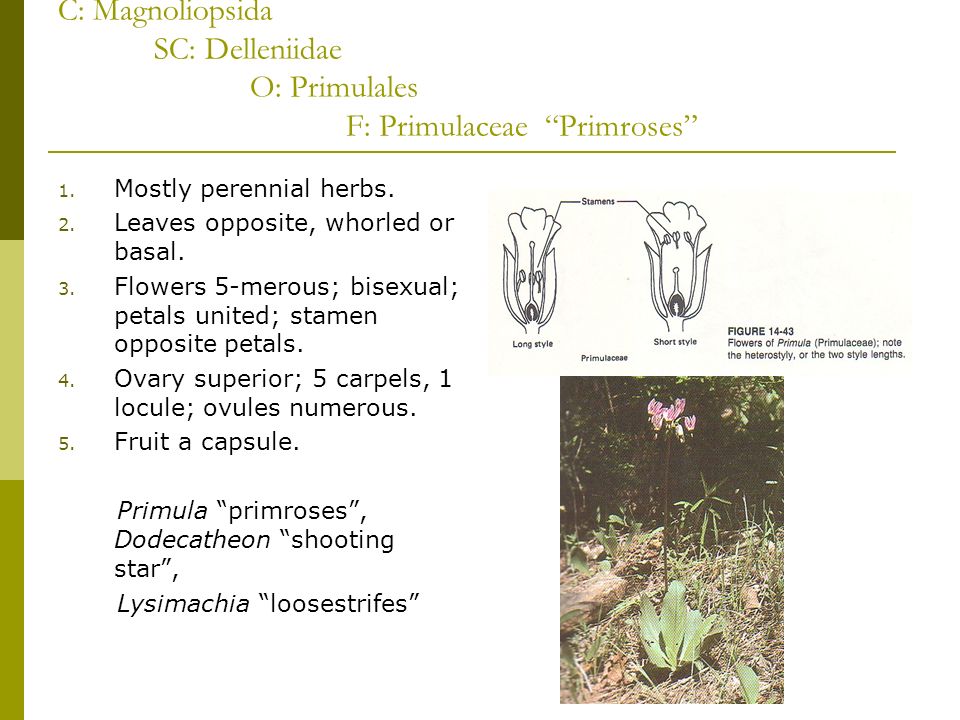The image appears to be a detailed page from a botanical book, showcasing a plant identified as a primrose. Dominating the bottom right corner is a faded photograph of the plant, which displays a thin brown stem bearing green leaves at the base and pink and white flowers at the top. A more precise botanical line drawing of the plant and its floral structures, including stamens, is located above the photograph. The text at the top of the page reads "C. Magnoliopsida, S.C. Delenidae, O. Primulales, F. Primulaceae, Primroses," indicating its scientific classification. The main body of the text includes a numbered list of characteristics: 1. Mostly perennial herbs; 2. Leaves opposite, whorled, or basal; 3. Flowers bisexual with united petals and stamens opposite the petals; 4. Superior ovary with five carpels; 5. Fruits in a capsule. Additional plant names such as Primula, Dodecathion (shooting star), and Lysimachia are mentioned. The left margin features a vertical gradient line transitioning from dark to bright green. At the top of the image, there is also a label reading, "Figure 14-43, Flowers of Primula, Primulaceae," with a note on the varying style lengths.